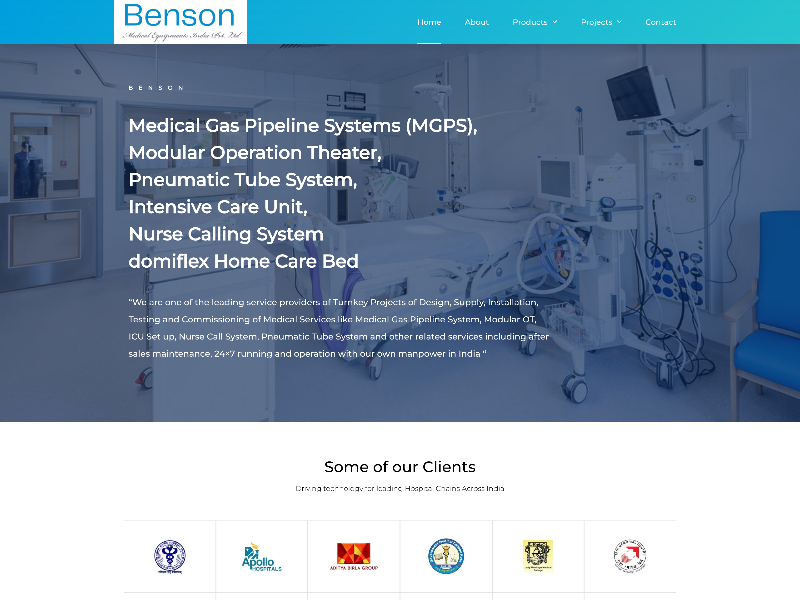The image shows a meticulously designed website interface. At the top, a striking turquoise blue banner spans across the width of the page, providing a vibrant header. Towards the left side of this banner, slightly inset from the edge, there is a distinct white rectangle that prominently displays "Benson and Capital" in the same turquoise blue font, emphasizing the company's branding.

Moving horizontally across the banner towards the right, a succinct navigation menu is neatly organized with the options: Home, About, Products, Projects, and Contact, allowing easy access to different sections of the website.

Beneath the banner, a hero image dominates the main content area. This image provides a glimpse into a hospital setting, showcasing a bed, a television, a monitor, and a nursing station. The image has a semi-transparent film overlay, giving it a subdued, faded appearance. 

Overlaying the top part of this background image, in crisp white text, there are the words "Benson" and directly below that, in bold, it states "Medical Gas Pipeline Systems (MGPS)." Additional services are listed underneath in the same bold print: "Modular Operation Theater, Pneumatic Tube System, Intensive Care Unit, Nurse Calling System, DomaFlex, Home Care Bed."

Further down the page, a section titled "Some of Our Clients" features six distinct squares, each containing a unique icon, symbolizing the various esteemed clients associated with the company. This clean, professional layout effectively communicates the diverse range of products and services offered by Benson and Capital.